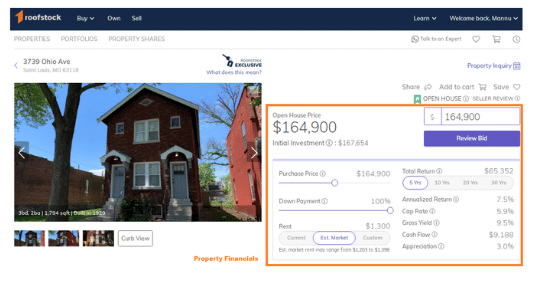A screenshot displays a real estate listing for what appears to be a townhouse. The exterior of the house is characterized by narrow, dark red brickwork. Prominently situated in the middle of the facade are two windows, one on the upper floor and one on the lower floor. Flanking the windows are two doors, one on each side. To the right of this house image, a red box highlights the financial details: the listed price is $164,900, with an initial investment of $167,654. The purchase price is reiterated as $164,900. Additionally, it highlights a down payment of 100%, and an expected rental income of $1,300 per month.